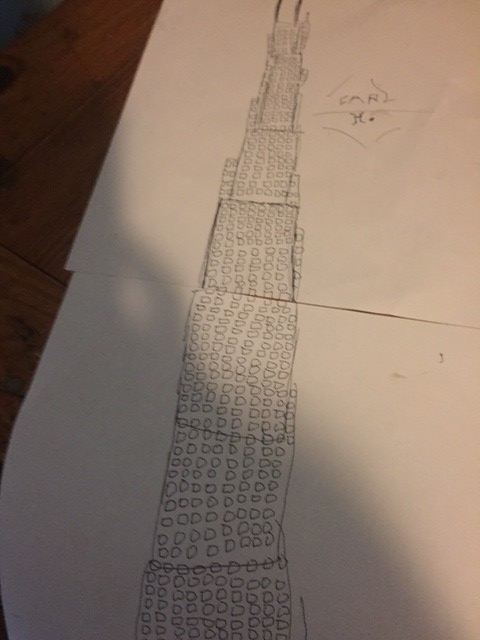This image is a photograph capturing a detailed pencil drawing composed on two separate sheets of paper, placed side by side. The drawing depicts an exceptionally tall building, characterized by its orderly grid of windows – approximately eight to ten windows per row, extending over an estimated one hundred rows. The building's substantial height is evident, with the bottom half of the structure illustrated on the lower sheet of paper, and the top, tapering slightly yet not culminating in a peak, on the upper sheet. A striking diagonal shadow crosses the lower portion of the building, adding depth and dimension to the otherwise uniformly rectangular edifice.

Adjacent to the main drawing, on the top sheet of paper, are additional pencil markings. These include an incomplete diamond shape intersected by a horizontal line, with what appears to be the letters "C-A-R" inscribed above. Beneath these letters lies a small, distinct symbol, also rendered in pencil.

The entire composition rests on a dark wooden surface, notable for its rich brown color and pronounced grain patterns, which provide a contrasting backdrop to the monochromatic sketch. This intricate scene, both in subject and background, creates a visually captivating study of architectural form and artistic intricacy.